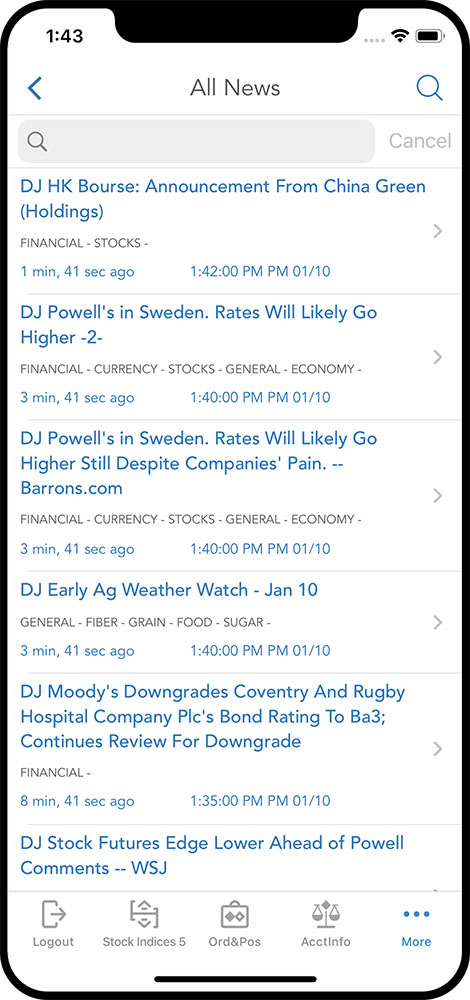The image is a detailed screenshot of a simulated smartphone interface, characterized by a sleek black border and a small black notch at the top, suggestive of contemporary phone designs. The display's backdrop is white, highlighted by black, blue, and gray fonts and icons. 

At the top of the screen, "143" is displayed in black. Adjacent to this are a Wi-Fi signal icon, a couple of gray circles, and a battery icon shaded in black. Below this status bar resides a blue arrow next to the text "All News." A gray search box containing a magnifying glass icon and the word "Cancel" in gray follows.

The central section of the screen features a prominent blue block showcasing various news headlines. The first headline reads, "DJHK Bourse announcement from China Green Holdings financial stocks," noted as being updated one minute and 41 seconds ago, at 1:42 p.m. on January 10th. Subsequent headlines provide timely financial news, such as:

- "DJ Powell's in Sweden. Rates will likely go higher to financial currency stocks. General economy," updated three minutes and 41 seconds ago at 1:40 p.m.
- "DJ early AG weather watch January 10th. General fiber grain food sugar," also updated three minutes and 41 seconds ago at 1:40 p.m.
- "DJ Moody's downgrades Coventry and Rugby Hospital Companies PLC's bond rating to BA3 continues review for downgrade," updated eight minutes and 41 seconds ago, at 1:35 p.m.
- "DJ stock futures edge lower ahead of Powell. Comments Wall Street Journal."

Towards the bottom of the screen, a white bar features several gray icons with labels such as:

- "Log out," accompanied by an icon of a paper with an arrow.
- "Stock indices," noted with an up and down arrow.
- "Order and POS," paired with a briefcase and diamonds icon.
- "Account info," symbolized by justice scales.
- "More," indicated by three blue circles.

A thin black line underlines this section, adding to the organized layout of the simulated phone interface.